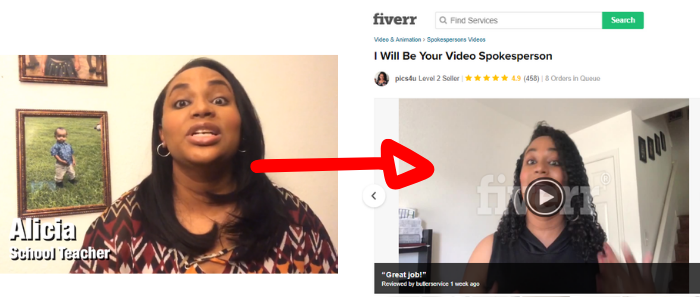In the side-by-side images, a black woman named Alicia is depicted standing against a wall adorned with family photos, possibly of a baby. She looks directly at the camera, with the caption identifying her as a school teacher. Adjacent to this, a second image labeled "5RR" (likely a gig work site) features the same woman. A red arrow connects the two images. On the "5RR" site, Alicia is presented as a video spokesperson with an accompanying play button for her video presentation. Below, a glowing review "Great job" endorses her services, and contact options are available for hiring her.